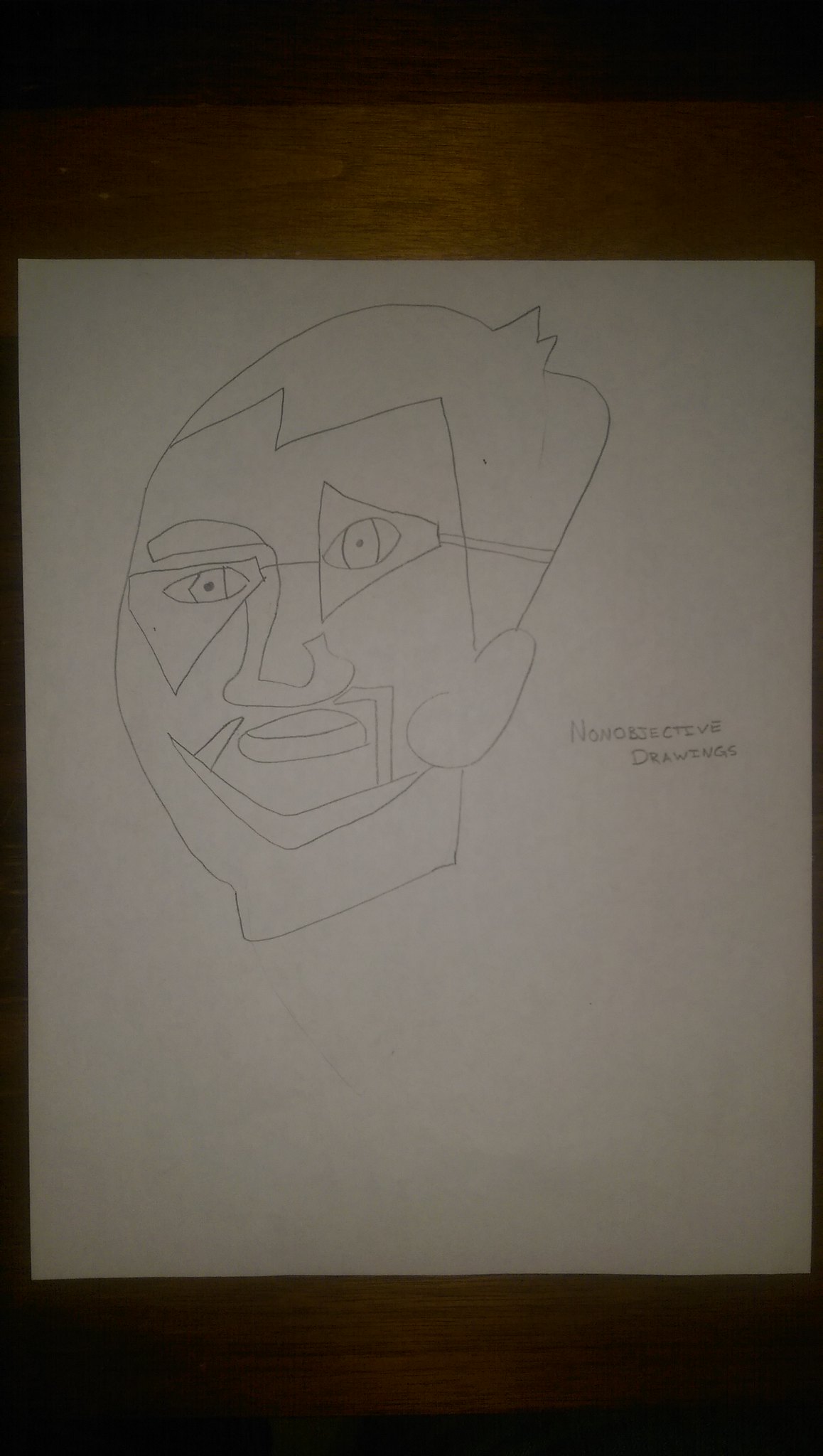This image depicts a drawing on a piece of printer paper, placed on a dark brown wooden desk. The drawing, likely done with a pencil as indicated by the presence of some erased lines, appears to be an abstract, Picasso-esque representation of a man's face, featuring an array of unconventional elements. The man's spiky, messy hair and triangular glasses, with the left lens facing outward and the right lens facing downward, add to the abstract quality. His face includes a single eyebrow connected to a nose that curls around, pursed lips, and an outline resembling a Van Gogh-style goatee, while the ear is unusually placed to the left of the goatee. The entire printer sheet is visible in the photograph, and next to the drawing, there is a handwritten note that seems to read "non-objective drawings." Despite being somewhat fuzzy and out of focus in a faded, dark photograph, the unique and abstract details of the drawing stand out distinctly.